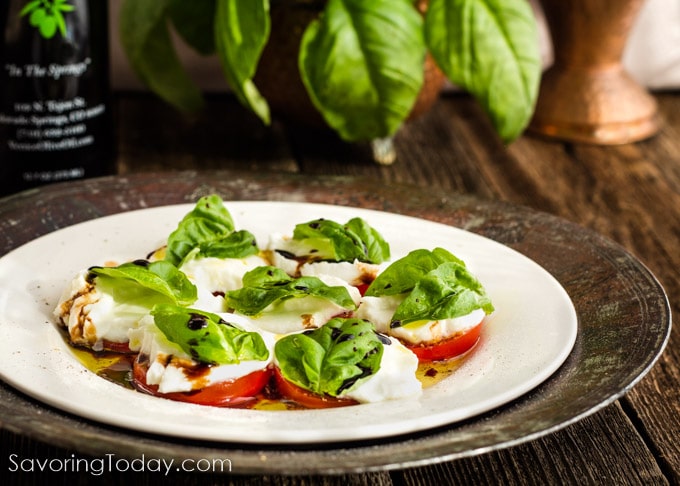The image is a detailed color photograph capturing a close-up of a beautifully arranged meal on a table. The scene features a shallow white ceramic plate set atop a rustic, aged, metallic brown plate. On the white plate, there are thick slices of juicy tomatoes, each layered with equally thick slices of melted white mozzarella cheese, partially burnt basil leaves, and drizzled with both olive oil and balsamic vinegar. In the background, a fresh basil plant, a dark wine-shaped bottle of olive oil, and a copper salt shaker add depth to the setting. The entire arrangement rests on a wooden table, and at the very bottom left corner, there's white text that reads "savoringtoday.com."